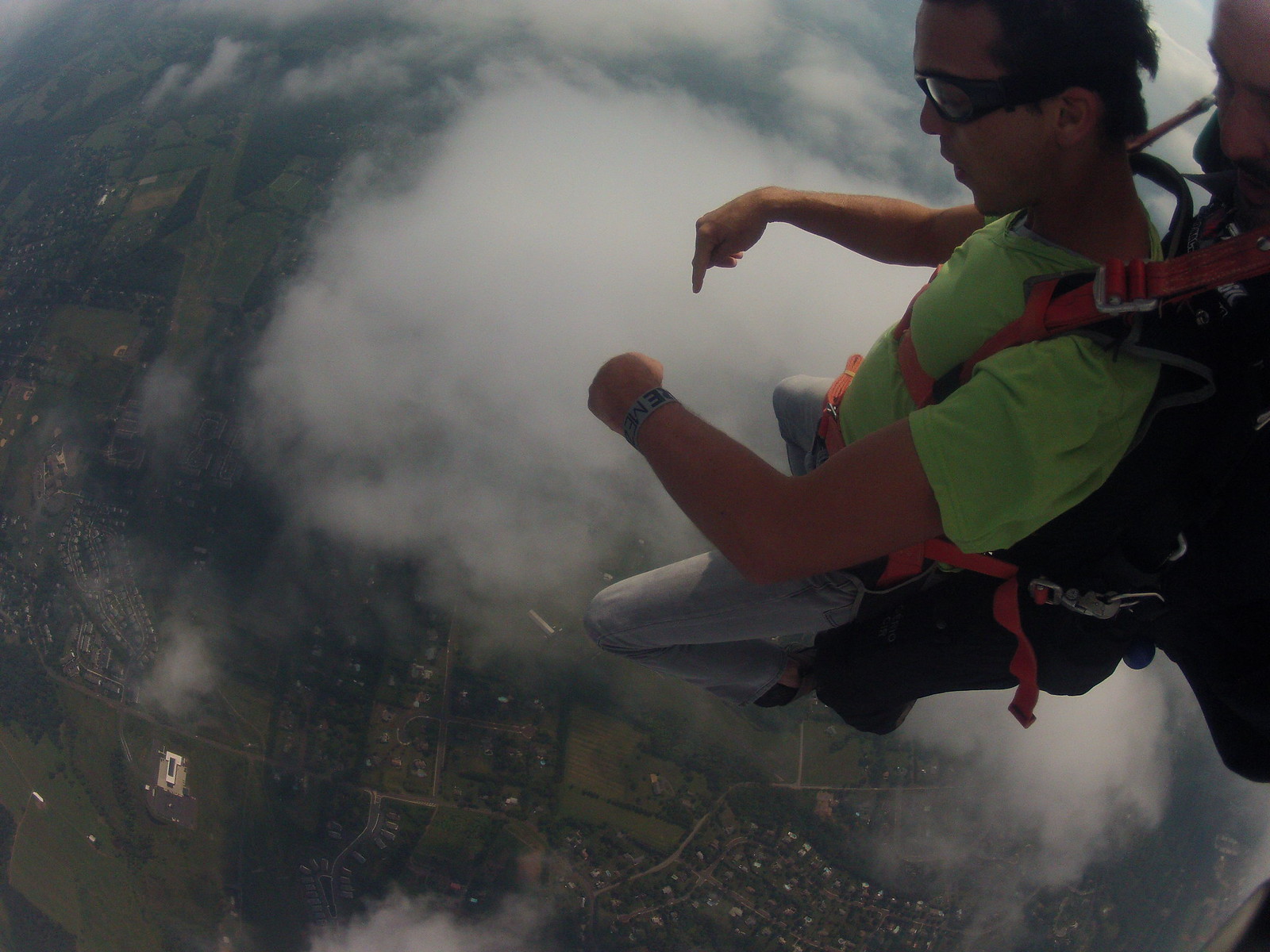This photograph captures a young male, most likely of Asian descent, tandem skydiving. He is dressed in a neon green t-shirt and distressed light blue jeans, with black Oakley sunglasses shielding his eyes and a cloth bracelet adorning his wrist. Beside him, a more experienced skydiver dressed in all black is securely attached with orange straps, guiding the descent. The young man is pointing downwards, his mouth shaped in an expression of awe, creating an "O" shape. The duo is high above the clouds, with a breathtaking view of tiny houses and expansive green fields below them. The image, possibly taken with a selfie stick, captures the adventurous moment just as they are about to or have just exited the airplane, with the clouds partially obstructing the earth below. The man’s expression, attire, and the setup suggest a thrilling skydive experience.